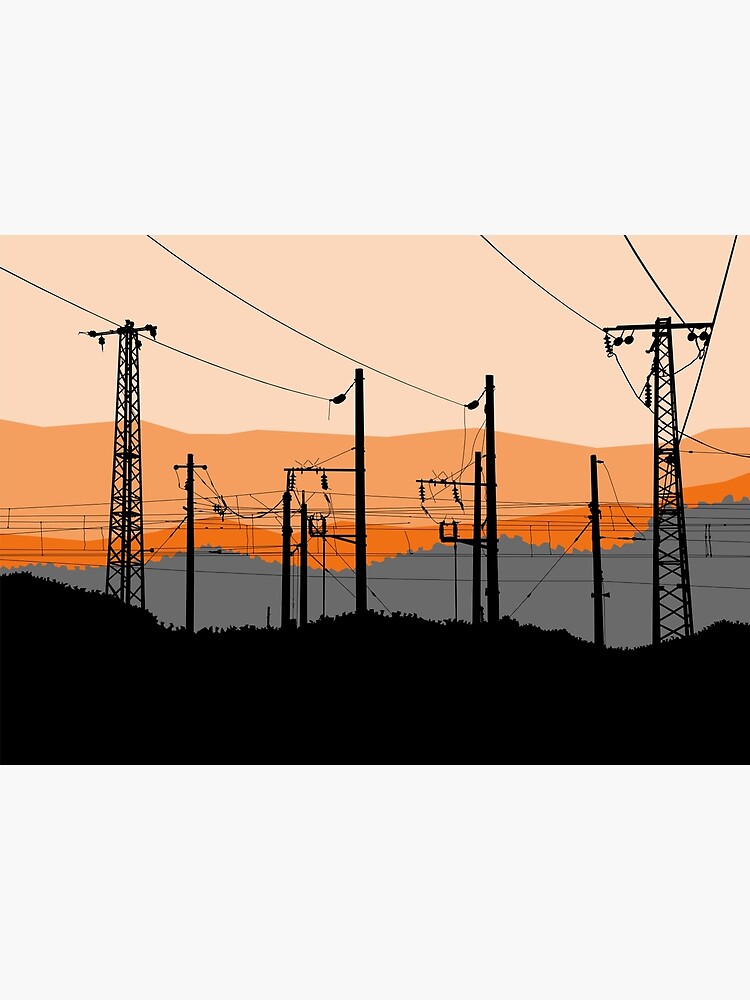This image is a detailed artwork depicting a remote area at either sunrise or sunset, featuring a network of power lines and power poles against a contrasting mountainous backdrop. The sky transitions from a pink hue at the top to an orange shade, meeting the blue-tinted representation of mountains beneath. The bottom third of the image is solid black, representing the ground. Prominently, two tall power poles stand on the left and right edges of the image, each with zig-zagging metal structures and numerous cables. Between them, there are four additional power poles in the center; the two outer ones are slightly shorter while the two inner poles vary in height. The lines connected to these poles crisscross in various directions, adding complexity to the scene. The digital-like quality of the image, with some pixelation visible, suggests it may be computer-generated, enhancing the surreal atmosphere of the desert-like landscape.